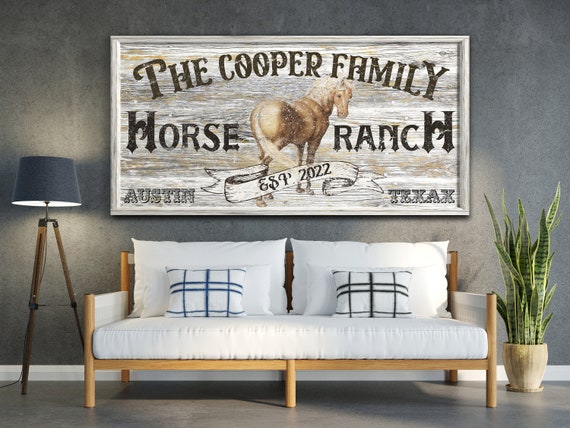In this modern living room, a striking, rustic wooden sign serves as the focal point, hanging prominently on a gray wall with white trim. The sign, encased in a bleached wood frame, proudly displays “The Cooper Family Horse Ranch, Austin, Texas, Established in 2022” in a Western font. At its center, a detailed depiction of a light brown horse with a blonde mane and tail adds a touch of charm. Below the sign sits a sleek, white couch framed in light wood, featuring a large white seat cushion, two matching back cushions, and accompanied by throw pillows—one with blue stripes and another with brown stripes. To the left of the couch stands a stylish tripod lamp with a blue lampshade, while a tall snake plant in a brown pot graces the right side, adding a splash of greenery to the scene. The room's decor is cohesively tied together with a grayish-brown floor, creating a warm and inviting atmosphere.